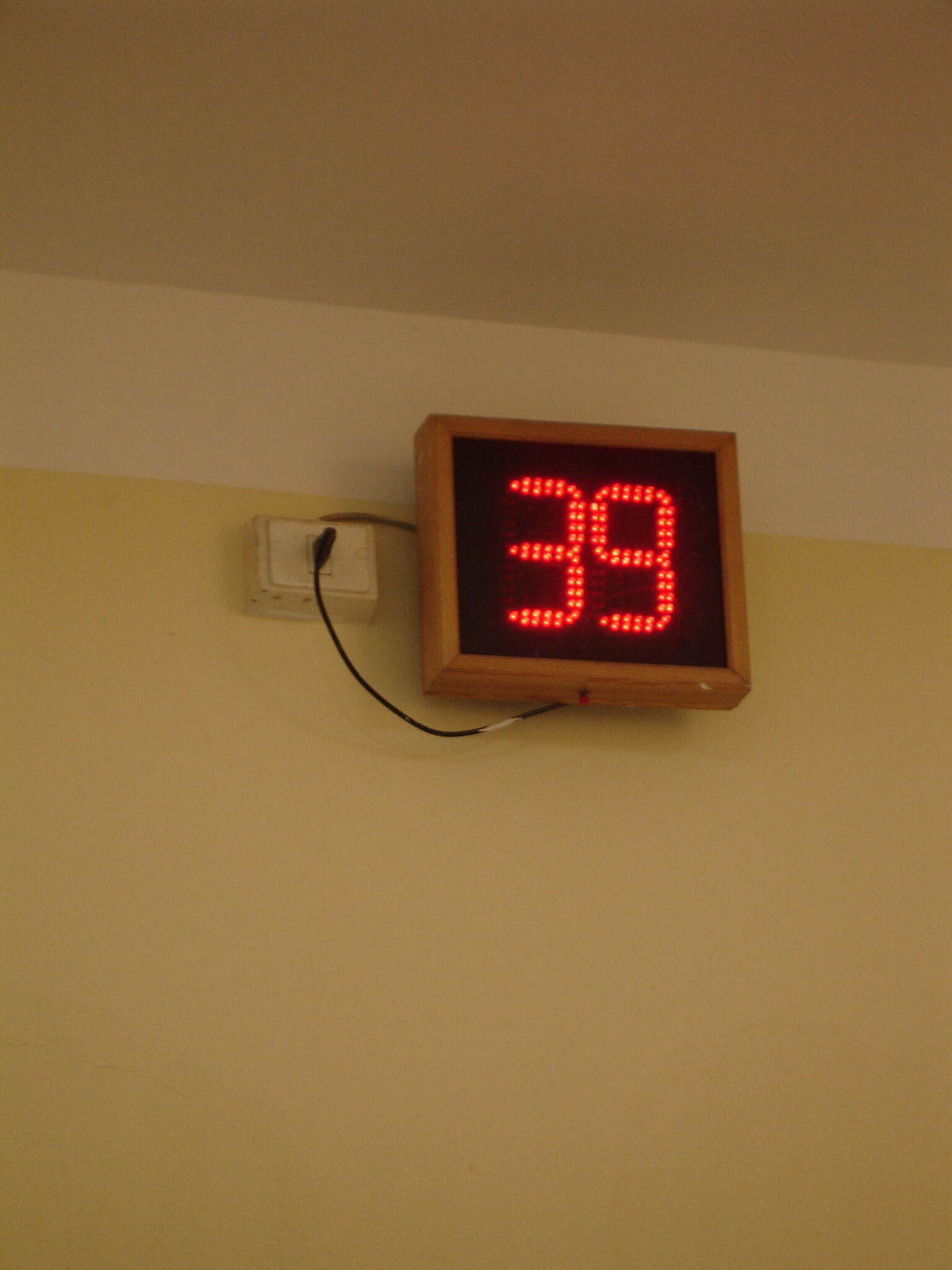This detailed image captures the juncture where a light yellow wall meets the ceiling. A strip of white trim highlights the top portion of the wall, seamlessly transitioning into the white ceiling above. Notably, affixed just below the ceiling, there is a square LED screen with a natural wood frame. The frame, crafted from light brown wood with visible darker wood grain, encloses the digital display, which shows the number "39" in bold red on a black background. Exiting the back of the screen, two wires are connected to a smaller white block mounted on the wall, resembling a phone jack rather than a conventional electrical outlet. The scene is set against a slightly grainy backdrop, suggesting a zoomed-in perspective. The LED screen and associated wiring cast subtle shadows, adding depth and realism to the composition.